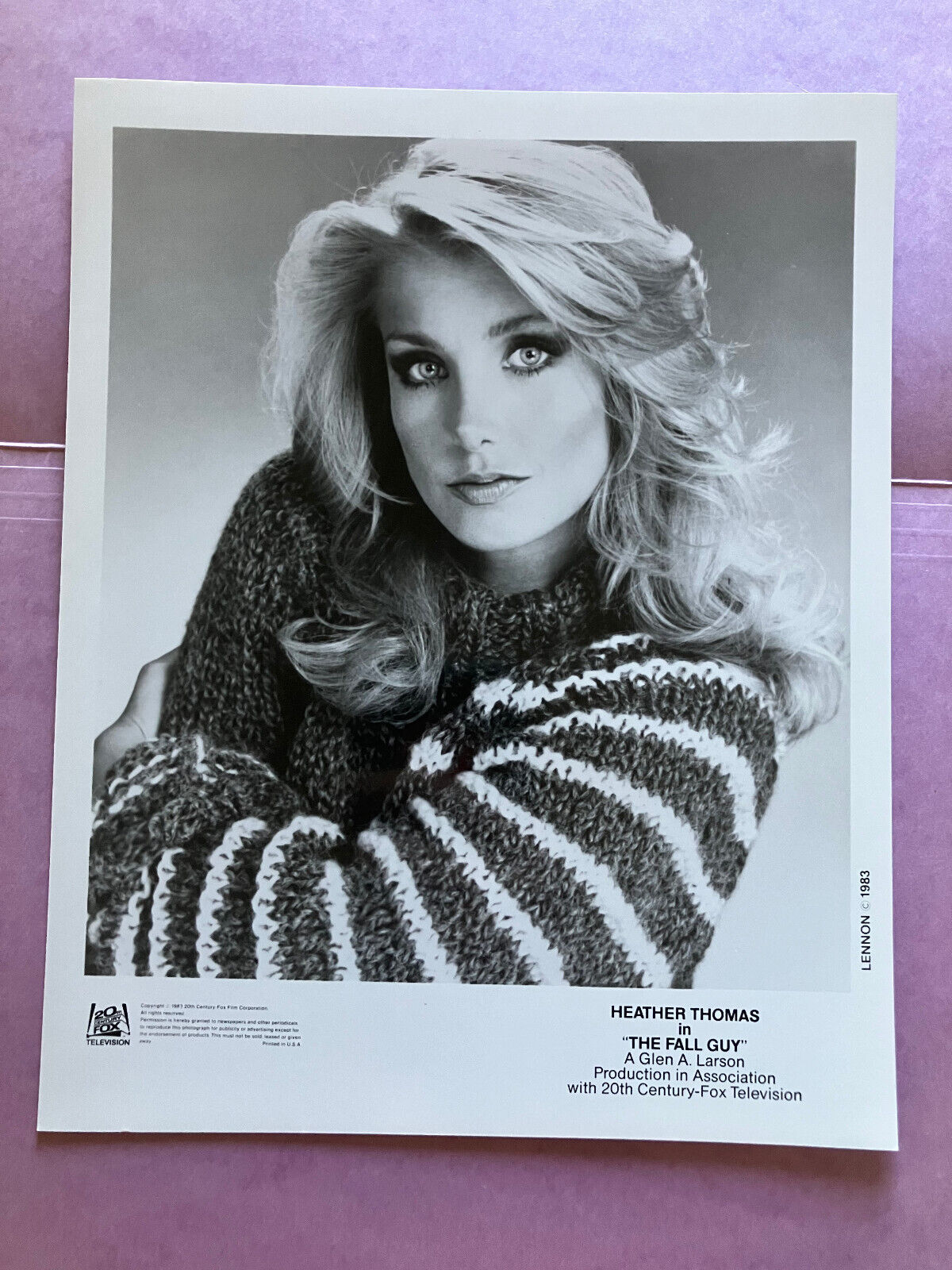This photograph, taken indoors, features an image set against a pink or possibly purple backdrop. It appears to be a black and white headshot of actress Heather Thomas, mounted on what looks like an 8.5x11 sheet of paper. Heather is depicted with long, wavy, blonde hair reminiscent of Farrah Fawcett's style, and her eyes, which are likely blue or green, are accentuated with thick, dark eye shadow. She is wearing a knitted sweater with distinctive horizontal white stripes down the sleeves. Heather's left arm is wrapped around her torso, with her hand gripping her right arm. At the bottom of the photo, bold black text reads, "Heather Thomas in 'The Fall Guy'," with smaller text underneath that says, “a Glenn A. Larson production in association with 20th Century Fox Television.” The photograph is copyrighted 1983, as indicated by some very small text and a logo on the left side, along with additional unreadable vertical text on the right side of the photo.